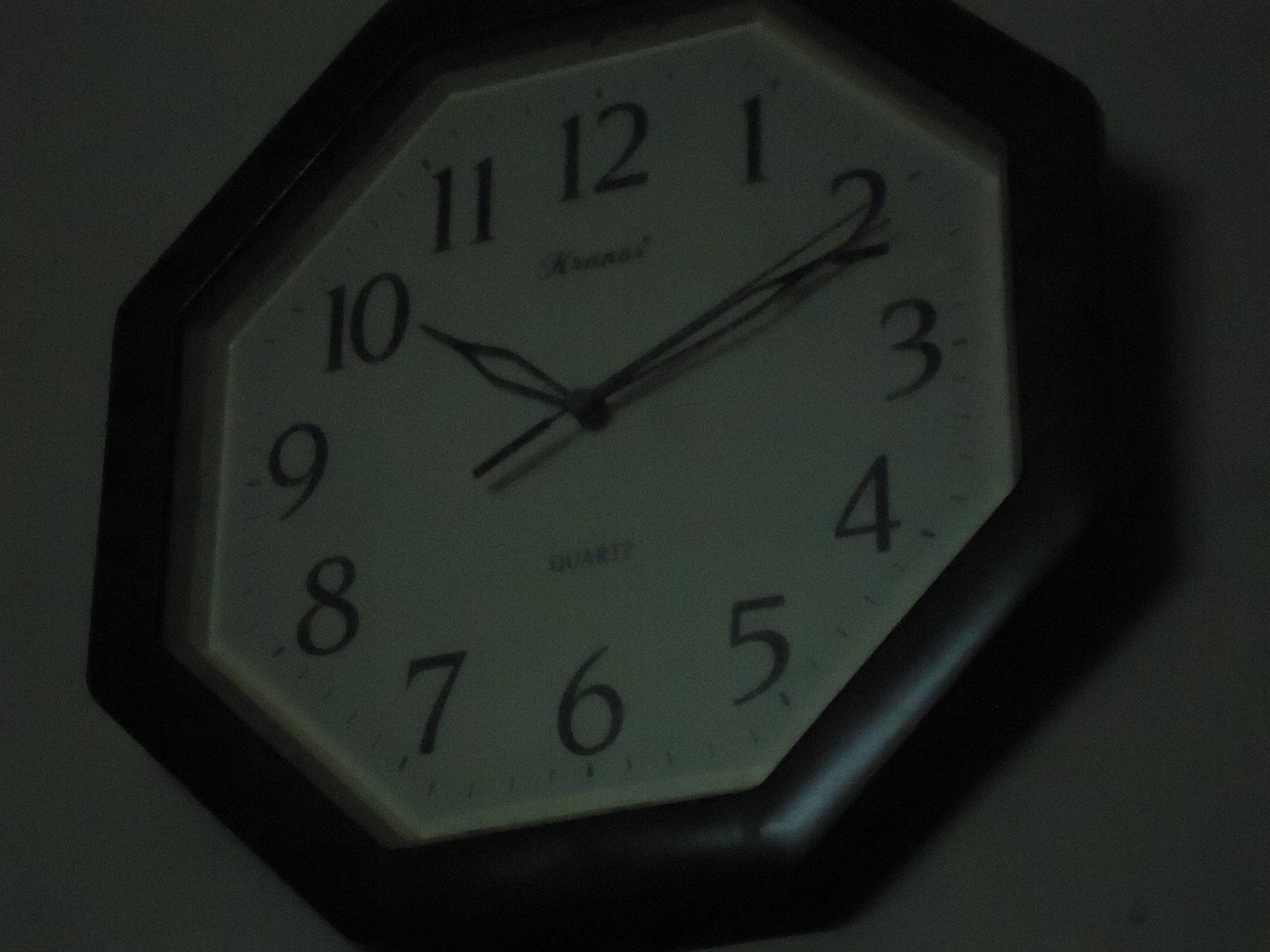This photograph depicts a clock mounted on a light gray, octagon-shaped wall. The image is quite dark, with minimal lighting highlighting the clock. The clock itself features a dark brown, geometric wooden frame and a white face. Black numbers, arranged from 1 to 12, are prominently displayed, with thinner dashes indicating the minutes. The clock reads approximately 10:10, with the second hand pointing near the 2. Subtle shadows cast by the clock's frame add depth to the scene. Beneath the number 12, faint text likely reads "quartz," though the dim lighting makes it difficult to discern the exact details.